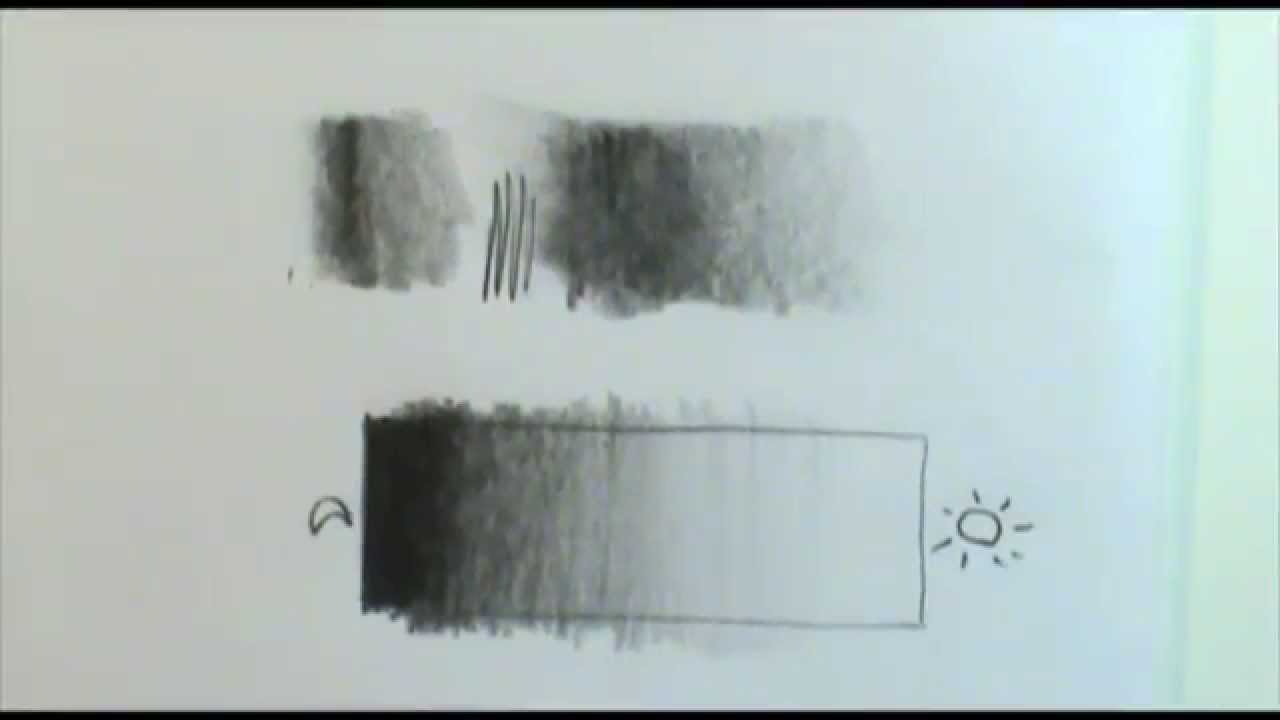The photograph, in landscape orientation with a black border at the top and bottom, depicts a child’s drawing on a partially visible light green wall. The main composition features two distinct sections. The upper part showcases a series of boxy scribbles with a pronounced zigzag line in the middle. Below this, a horizontal rectangle is meticulously outlined. Within this rectangle, on the left, a crescent moon is drawn, resembling a smiling mouth, while on the right side, there is a depiction of the sun, characterized by a circular shape with small specks suggesting rays. The interior of the rectangle transitions from a dark shade of black on the left, gradually lightening to white towards the right. The color wash and the gradient add a dynamic visual effect, enhancing the contrast between the dark and light areas. Overall, the artwork emanates a sense of balance and transition from night to day.